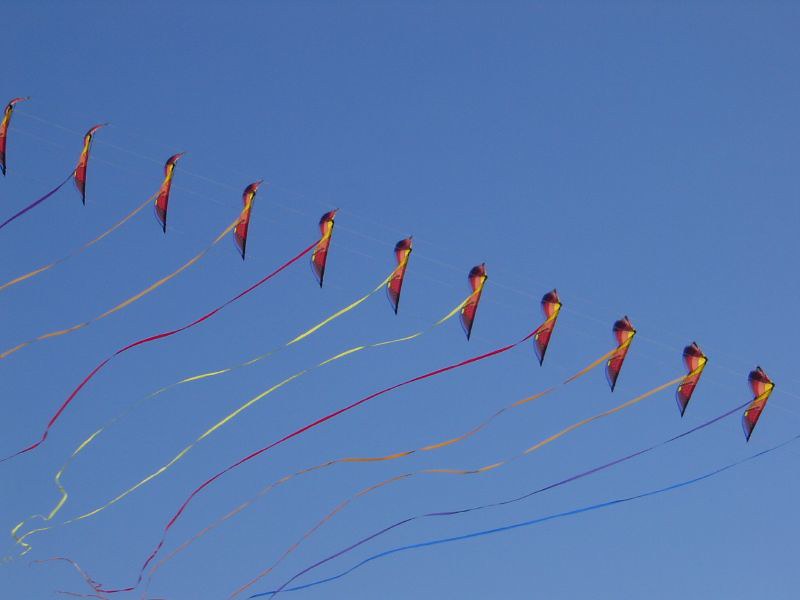The image captures a vibrant, cloudless blue sky filled with a string of connected kites, each exhibiting a radiant array of colors including red, orange, yellow, purple, and blue. The kites, which number approximately eleven, are arranged in a horizontal row with an unusual shape, wider at the top and narrower at the bottom. Each kite is adorned with tassels and individually colored strings that trail behind them, fluttering vigorously in the wind. The strings behind each kite are a visual spectacle of blue, yellow, red, and other hues, perfectly complementing the pristine day, suggesting ideal conditions for kite flying.